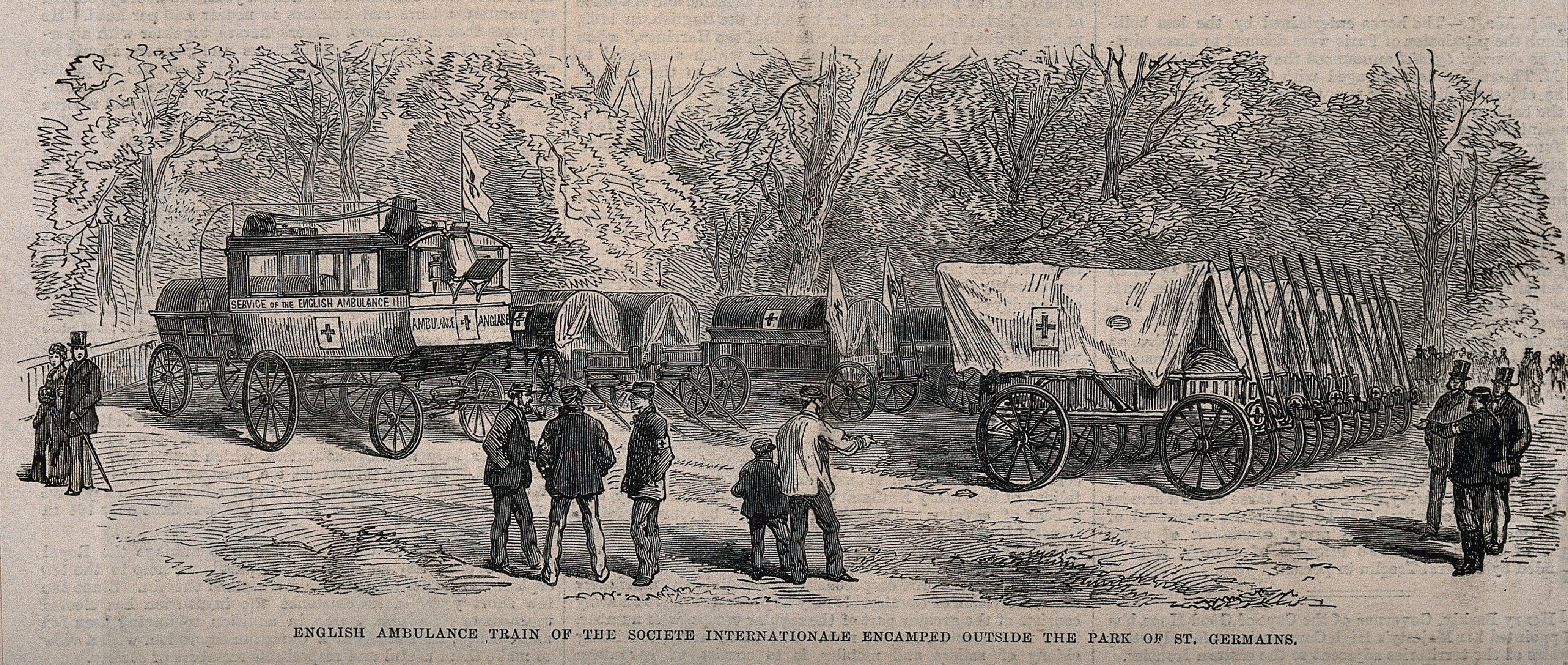This detailed vintage artist sketch portrays the English ambulance train of the Society International encamped outside the park of St. Germain. The scene features numerous horse-drawn ambulances, resembling enclosed carriages and Conestoga-style wagons with tarpaulin-covered frames. Each wagon prominently displays a cross emblem. In the background, meticulously sketched old-growth trees and park-like groves add depth to the setting. To the left, a gentleman in a high-top hat and a lady in traditional clothing stand alongside a young boy who seems to be assisting the ambulance corps. The right side of the image includes more gentlemen in high-top hats, soldiers with flat caps, and other figures. The black-and-white depiction, rendered in a variety of line directions and shadows, evokes a historic era with groups of people mingling in front of the ambulance trains. The ground beneath them is shaded with intricate details, reinforcing the image's antiquated ambiance.